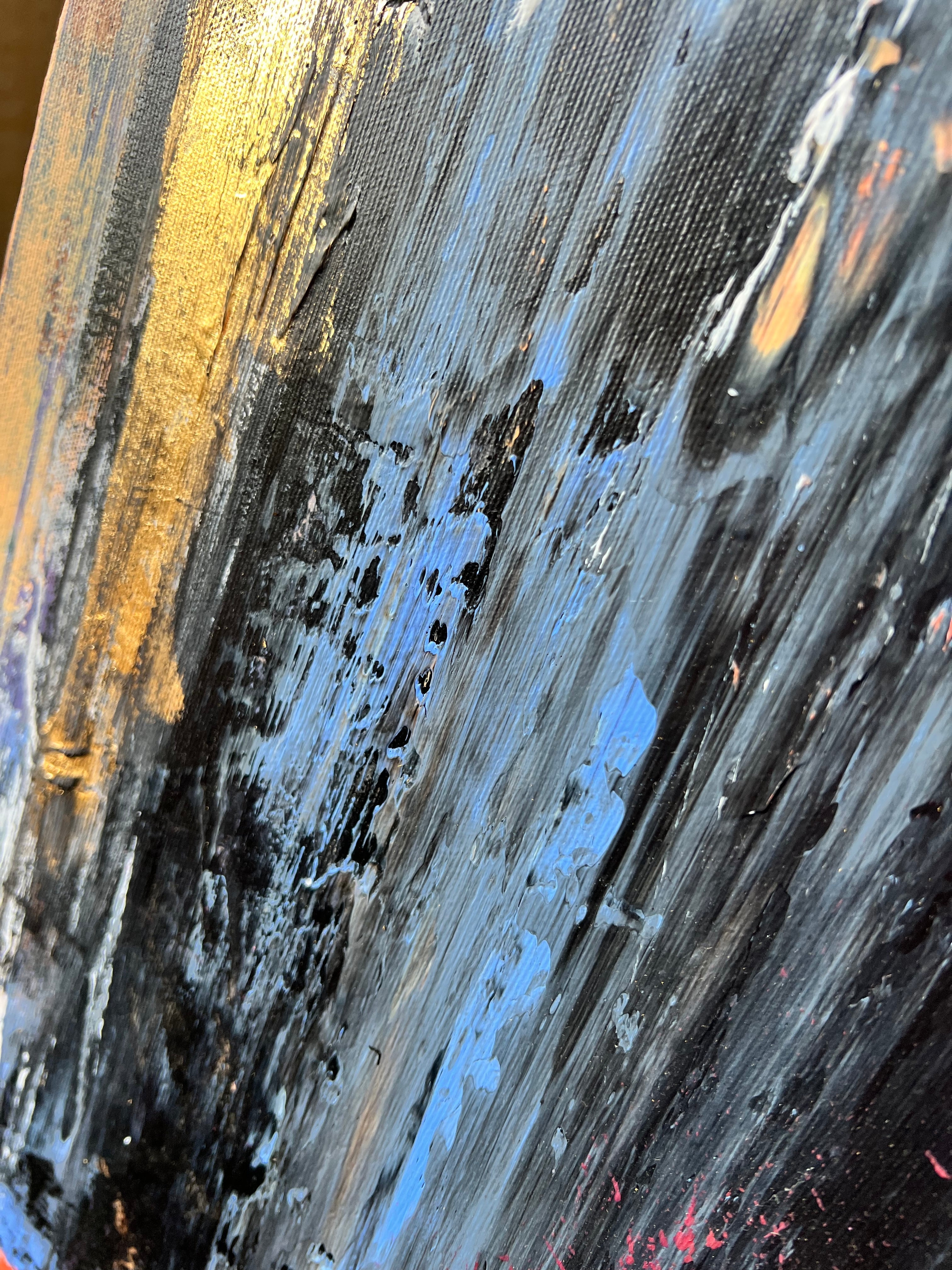The image showcases an abstract painting characterized by a dynamic interplay of colors and textures. Predominantly featuring vertical and diagonal striping, the colors transition fluidly across the canvas. Starting from the left, the color palette includes lighter hues such as peach, light gray, and yellow, which gradually darken into deeper shades of blue, gray, and black towards the center. Notably, the painting begins with a hint of darker orange and a dominant goldish hue at the upper left corner. The right side of the image is marked by more intense and smudged colors, including yellows, orange-gold, and various grays blending into each other. The texture of the canvas is visible beneath the paint, adding a tactile dimension to the artwork. Additionally, the bottom right corner features tiny pink splatters, creating subtle focal points against the predominantly darker background. The entire piece conveys an intricate balance of colors and a sense of movement, inviting viewers to explore its abstract complexity.